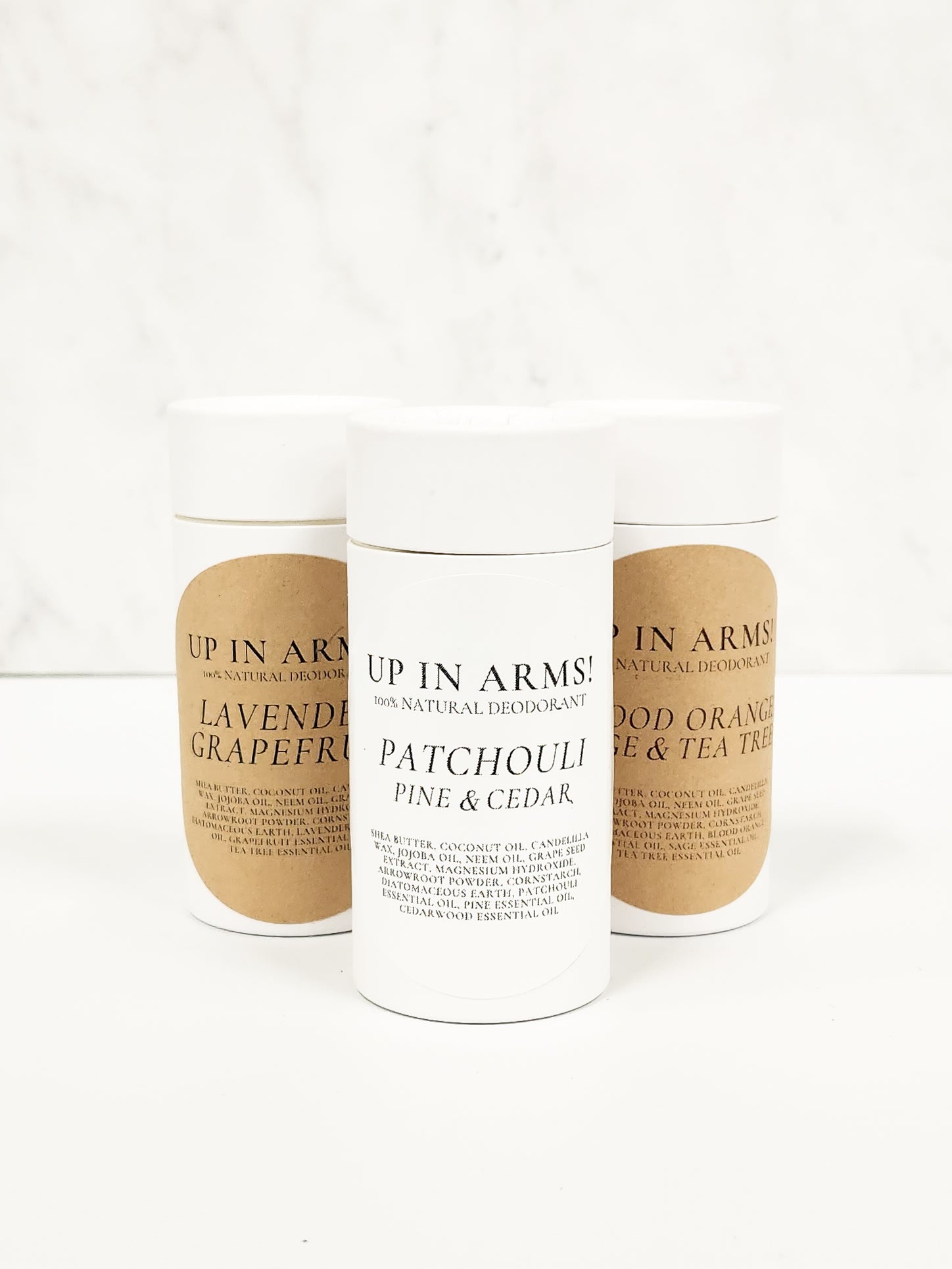The image depicts three containers of "Up In Arms" 100% natural deodorant, positioned on a clear or white surface with a white background that has subtle texture. The containers are arranged in a triangular formation, with the middle one slightly forward. Each container features a distinct label: the leftmost and rightmost labels are brown, while the middle label is white. The left container is labeled "Lavender Grapefruit," the middle container is labeled "Patchouli Pine and Cedar," and the right container reads "Blood Orange and Tea Tree." Highlighted ingredients on the labels include shea butter, coconut oil, candelilla wax, jojoba oil, neem oil, grapeseed extract, magnesium hydroxide, arrowroot powder, cornstarch, diatomaceous earth, essential oils, and additional natural scents corresponding to each variety.